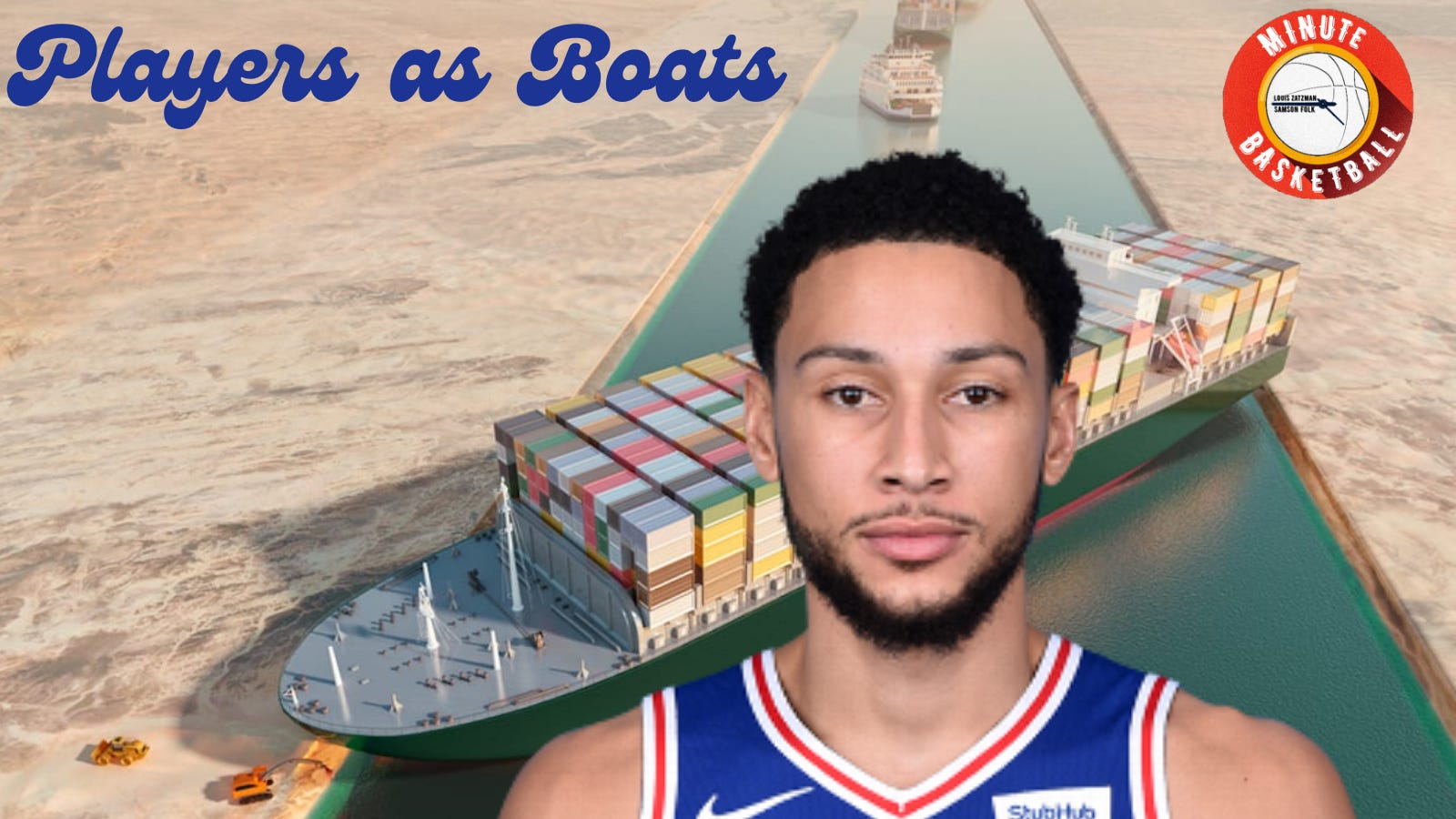This image portrays an African-American basketball player with a light complexion, a beard, mustache, and short curly hair. He is adorned in a blue basketball jersey outlined with red and white stripes, featuring a Nike symbol on one side and a StubHub patch on the other. The jersey is styled like a tank top with a V-neck, typical of basketball attire. The top left corner of the image reads "Players as Boats," while the top right corner displays "Minute Basketball" in a red circle with a basketball icon in the center. The background depicts a canal flanked by desert terrain, containing cargo ships loaded with storage containers. One ship is prominently stuck mid-canal, with additional vessels visible behind it. The player gazes directly at the viewer, situated in the forefront of this dynamic and likely advertisement-themed scene.